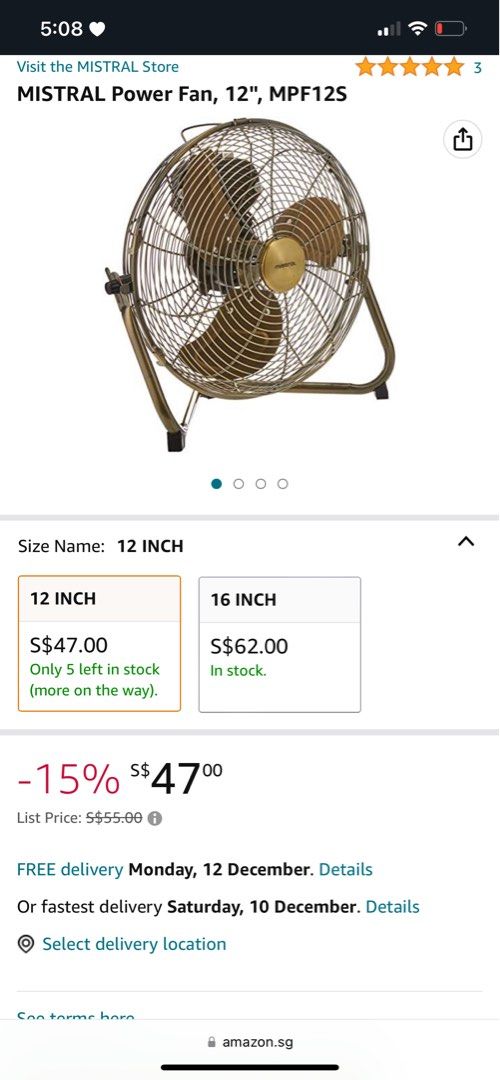The image features a Mistral Power Fan available for sale, model MPF123. The primary fan in the picture is a 12-inch version priced at $47, with an indication that only five units are left in stock, though more are on the way. The image also highlights that there is a larger, 16-inch version priced at $62 which is currently in stock. A promotional red text shows a 15% discount on the 12-inch fan, confirming its price as $47. 

At the top of the image, there is a clickable section that says "Visit the Mistral Store," which promises more information. This section shows one active blue dot with three additional dots, suggesting the availability of three more images to view. 

Under the fan's pricing details, there is an option for free delivery by Monday, December 12th, or faster delivery by Saturday, December 10th. Additionally, two blue clickable links are available for further interactions: one labeled "Details" and another labeled "Select Delivery Location."